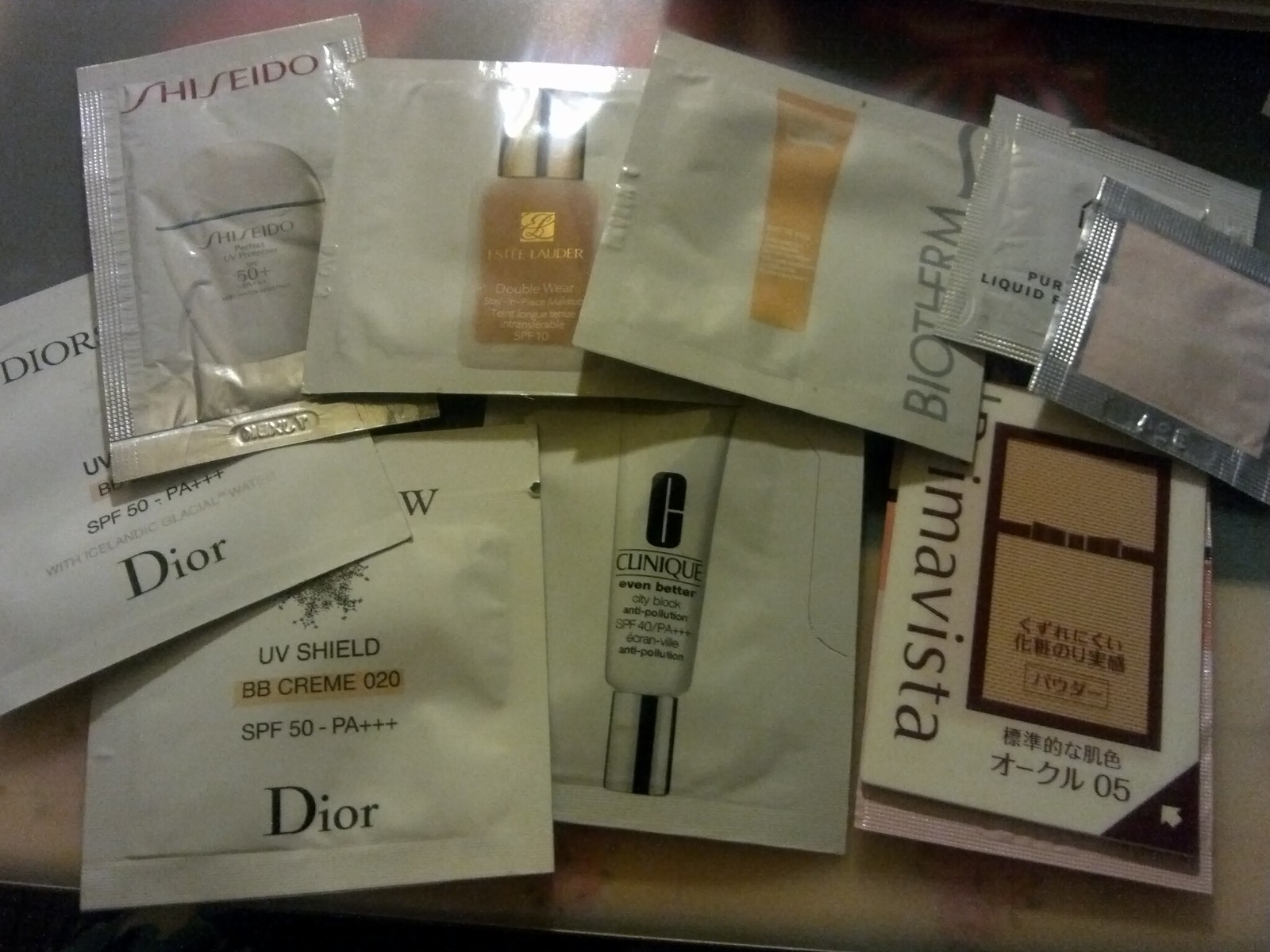An indoor, color, close-up photograph captures a bird's-eye view of a wooden table adorned with a collection of nine small perfume sample packets. The packets are meticulously arranged in two overlapping rows: the top row containing six packets and the bottom row comprising three. Each packet is flat, square-shaped, and predominantly white.

Starting from the left in the top row, the first packet bears the word "you're" at the bottom. Adjacent to it, slightly overlapping, is a packet labeled "SHISEIDO" at the top. Next, moving toward the center, there is a packet with an image of a clear glass perfume bottle filled with a golden liquid, although the text on it is not legible. Continuing to the right, another packet features an image of a yellow liquid-filled tube with a white cap, oriented with the cap pointing downward, branded "BIOTHERM" vertically on the right side. Near the right edge of the top row are two smaller square packets; one is white, while the one overlapping it is silver with a pink center.

In the bottom row, the leftmost packet has the word "DIOR" printed at the bottom. Positioned centrally beneath this packet is another packet showing a white tube with a silver cap, oriented with the cap pointing downwards and marked "CLINIQUE" in black letters. Completing the arrangement, the rightmost packet in the bottom row is rectangular with a white label featuring a brown rectangle in the center, adorned with some Asian characters.